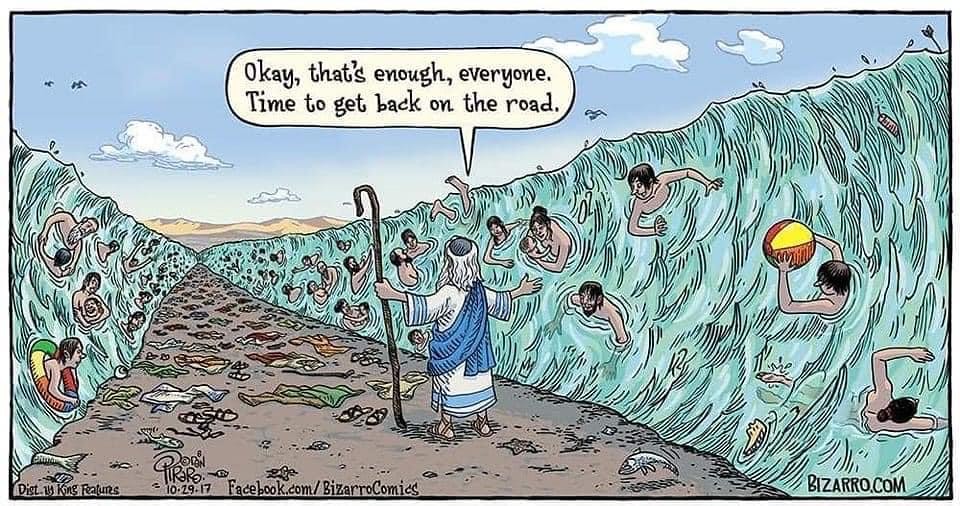The comic illustration depicts a humorous and anachronistic scene of Moses parting the Red Sea. Moses, identifiable by his white robe, blue sash, sandals, gray hair, and yarmulke, stands in the foreground with his arms outstretched, holding a long, looped walking stick in his left hand. He speaks through a white speech bubble that reads, "Okay, that's enough everyone. Time to get back on the road." The parted sea reveals a sandy path strewn with various articles of clothing, sandals, and a few dead fish, as if left behind by those crossing. On either side, the walls of water are filled with men, women, and children enjoying a swim, with some using a beach ball and a float. Above the scene, the sky is depicted with birds, scattered clouds, and distant mountains. The bottom corners of the comic indicate the artist's website, bizarro.com, and a date, 102917, along with facebook.com/bizarrocomics.